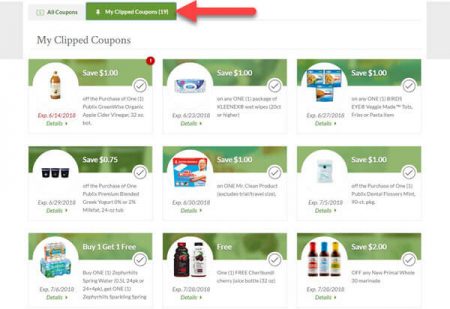The image depicts a webpage from a coupon website, specifically showing the "My Clipped Coupons" section. At the top of the page, there's a red arrow pointing to a button labeled "My Clipped Coupons," which is adjacent to another button named "All Coupons." There are nine clipped coupons displayed in a list format, each with specific details and potential savings. The coupons listed are as follows:

1. **Apple Cider Vinegar** - Save $1.
2. **Kleenex Wet Wipes** - Save $1.
3. **Veggie Made Tots or Fries** - Save $1.
4. **Greek Yogurt** - Save $0.75.
5. **Mr. Clean Products** - Save $1.
6. **Dental Flossers** - Save $1.
7. **Spring Water (Sparkling)** - Buy One Get One Free.
8. **Cherry Juice Bottle** - Free.
9. **New Primal Marinades** - Save $2.

Each coupon includes an expiration date, and users can click on the coupons to view more details, including usage restrictions and additional terms. The coupons displayed are the ones that the user has clipped and intends to use, either during their shopping trips or before the coupons expire.